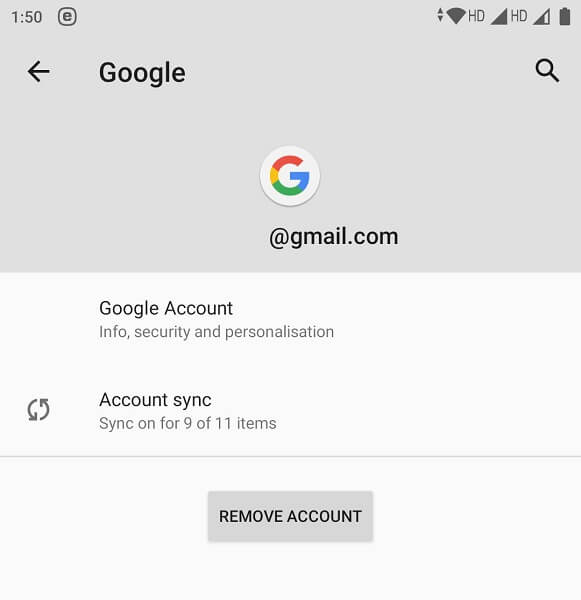This screenshot captures a section of a smartphone screen at 1:50, as indicated by the time display at the top. The screen is connected to Wi-Fi, with the battery level and network coverage icons visible. The left side of the screen header features a left-pointing arrow next to the word "Google," while a magnifying glass symbolizing the search icon is on the right. Below this, the familiar multicolored "G" Google logo is displayed within a white circle. Beneath the logo, the text "gmail.com" appears, followed by menu options such as "Google Account," "info," "security," and "personalization." Additionally, the screen shows that account synchronization is active for 9 out of 11 items. At the bottom, a gray rectangle features the option "Remove account" in black lettering. The image is devoid of any photographic elements, people, animals, birds, plants, flowers, trees, buildings, signs, billboards, flags, banners, mountains, or automobiles.